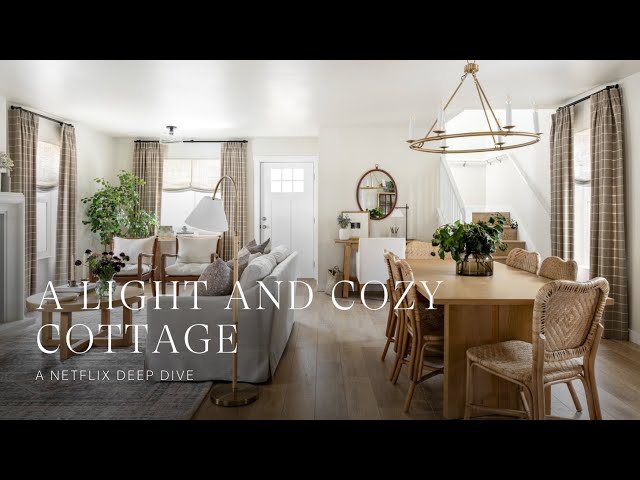The image is a title page for a Netflix show titled, "A Light and Cozy Cottage: A Netflix Deep Dive," as indicated by the white text on the left side. The setting is an inviting and warm living room and dining room area. The room has wooden floors and is adorned with a grayish white area rug. Central to the living room is a brown coffee table topped with a green plant and purple flowers, accompanied by a white couch and two additional small chairs. The room features three windows adorned with brownish drapes and has a white door positioned at the center-back.

Off the rug, the dining area features a wooden table with a green plant as its centerpiece, surrounded by five wicker chairs in a brown hue. The dining space is illuminated by a charming brownish-golden chandelier that hangs above the table. Additional elements include a mirror against the back wall, where a small wooden table and a white chair are positioned.

Overall, the cozy setting includes multiple plants, a brown plaid curtain on the right, and various lighting elements like lamps and candelabras, contributing to the room's warm and inviting atmosphere.